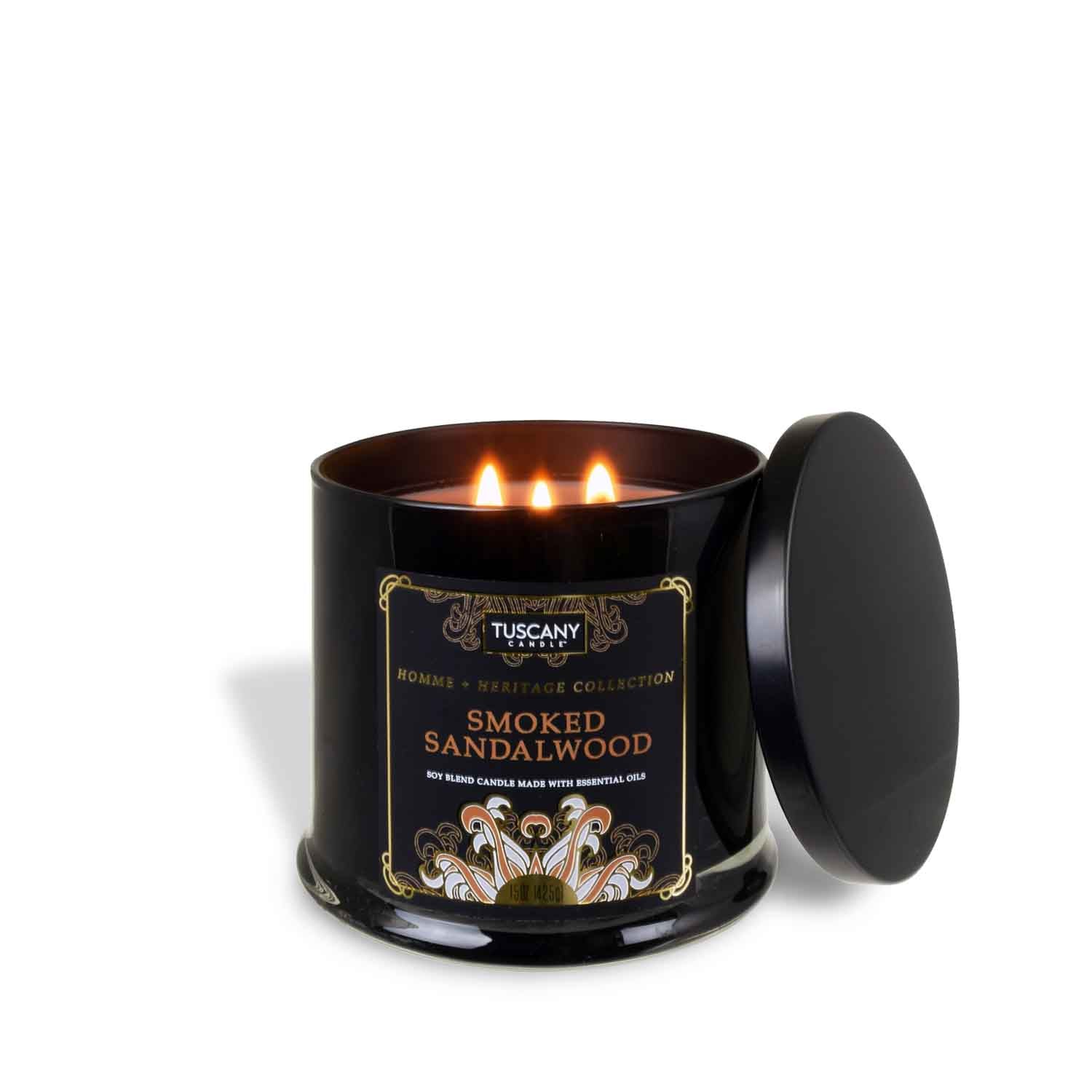The photograph is a highly detailed, square-format color image featuring a decorative scented candle as its central subject. The candle, which has a light tannish-pink wax and three burning wicks, is housed in a round, shiny black tin container with a slightly fluted bottom, adding to its elegance. The lid, matching in the same black finish, is propped against the container to the right. A label adorns the front of the tin, bordered by a shiny gold metallic outline with decorative corner flourishes. The label details include a black horizontal rectangle with white text reading "Tuscany Candle" at the top center, accompanied by smaller gold lettering that says "HOME. HERITAGE COLLECTION." Below this, in larger orange text, is the scent description, "Smoked Sandalwood." Additional white text at the bottom specifies that it’s a soy blend candle made with essential oils. Adding a touch of artistry, the bottom of the label features a peachy-orange and white swirling design. The candle’s flames flicker against an otherwise white, minimalist background with a subtle shadow cast behind both the tin and the lid, exemplifying photographic representationalism realism in product photography.